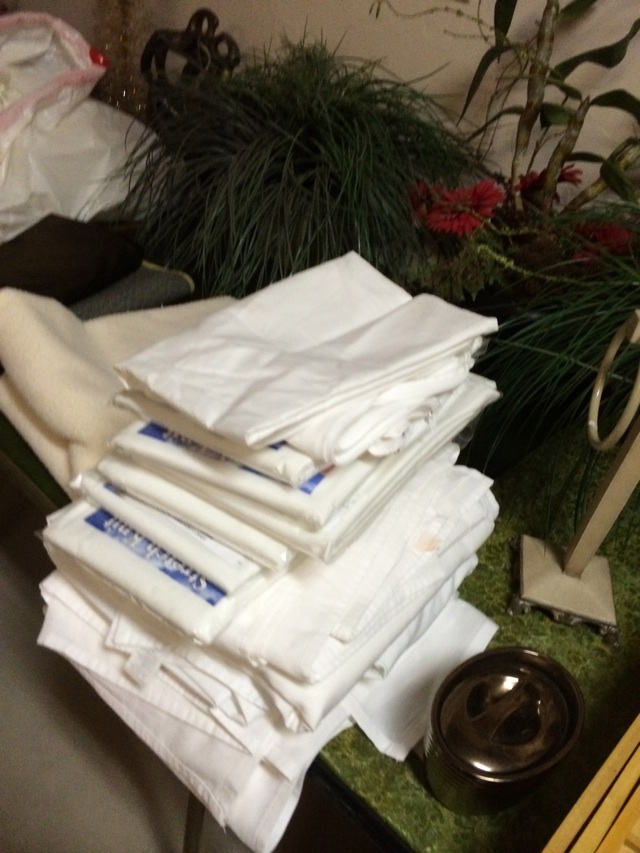The photograph depicts a stack of folded white linens that are prominently displayed on a jade green tabletop. These linens, some of which are still in their packaging with a blue label, appear to be freshly laundered tablecloths or handkerchiefs. The stack is quite high, with the topmost items having a smooth texture, while the bottom ones seem to have a terrycloth texture. To the left of this main stack, there is a larger, cream-colored tablecloth, a black piece of fabric, and a white trash bag placed on top of it. On the right side of the image, there is a black or dark gray lid, which seems like it belongs to a container, and further up, there is a squared dark gray base with an attached light gray rectangular beam that has a small ring, resembling a towel rack. In the background, a variety of indoor plants are visible, including long, skinny green blades of grass, regular green leafy plants, and some featuring red or pink flowers, all set against a white wall.